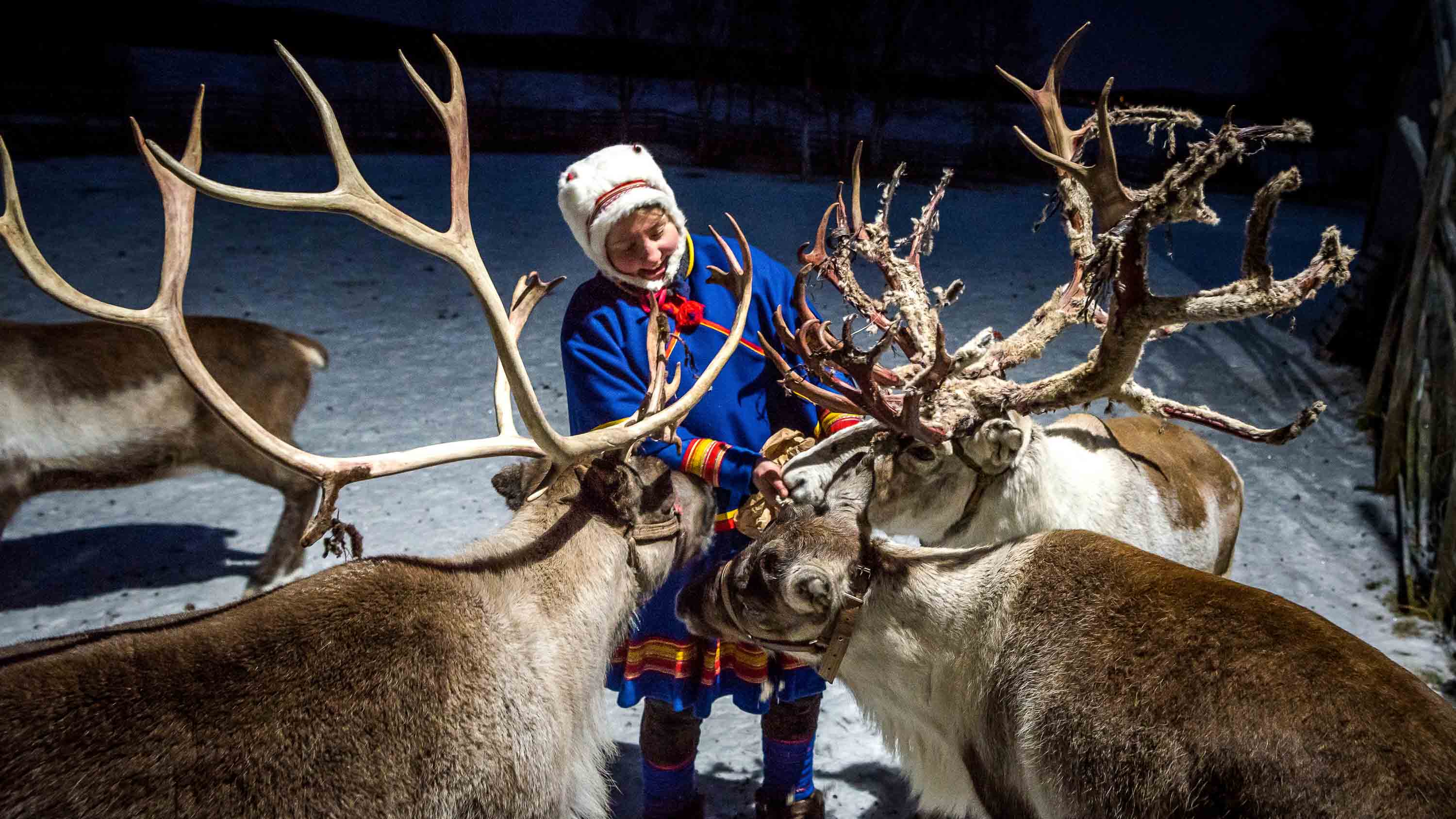In the image, a woman with a light complexion is standing outside at nighttime, surrounded by four moose in a snowy landscape. She is wearing a white fur hat and a blue coat that reaches her knees, adorned with colorful red and white stripes at the hem and sleeves, and bands of yellow and red around the middle. Her coat also has a tassel at the neck. The woman, who appears to have curly hair but her face is downcast, is feeding the moose as they gather closely around her. Some moose seem to have partially shed antlers, while others have fully grown ones, and they are fitted with harnesses, indicating they might be domesticated. The scene is illuminated by artificial light, making the woman and the moose clearly visible against the dark, tree-dotted background. The overall atmosphere suggests a serene and joyful interaction between the woman and the moose amidst the tranquil, snowy night.